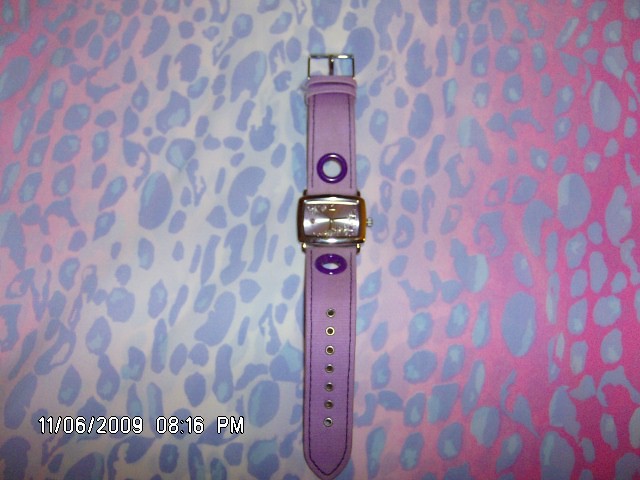A photograph captures a stylish rectangular watch resting on a vividly patterned background, likely a sheet or pillowcase. The background features an eye-catching leopard print in a gradient that transitions from hot pink to purple to light blue, then back to pink and hot pink. The watch's face is a sleek metallic lavender, harmonizing with its lavender bands which each feature a dark purple circle above and below the watch face. A digital time stamp in the bottom left corner reads "11-06-2009" and "8:16 PM," indicating the photo was taken on November 6, 2009, at 8:16 PM, most likely using a digital camera.